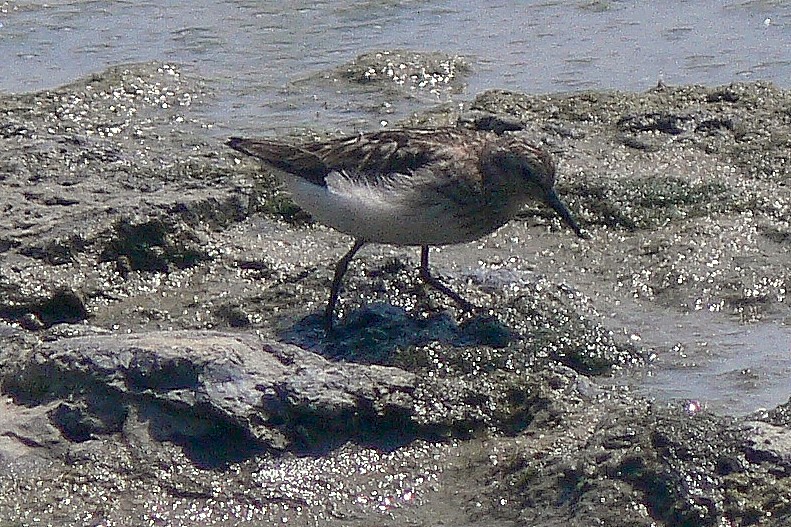This landscape-oriented photograph, taken during the daytime at a downward angle, features a small water bird, likely a type of sandpiper, positioned centrally. The bird stands on two legs near a muddy, rocky waterline with a puddle of water in front and a larger body of murky, grayish water behind. The surroundings include gray rocks mixed with small white shells or rocks. The bird, depicted in a close-up, has a dark brown back and a white underbelly, with legs and a long beak that appear dark black or brown. Its wings, folded against its body, are white, and it has a short tail. The bird is captured in profile, walking towards the right, with its beak pointed downward towards the puddle. The scene conveys a natural, outdoor setting in a detailed and realistic style.